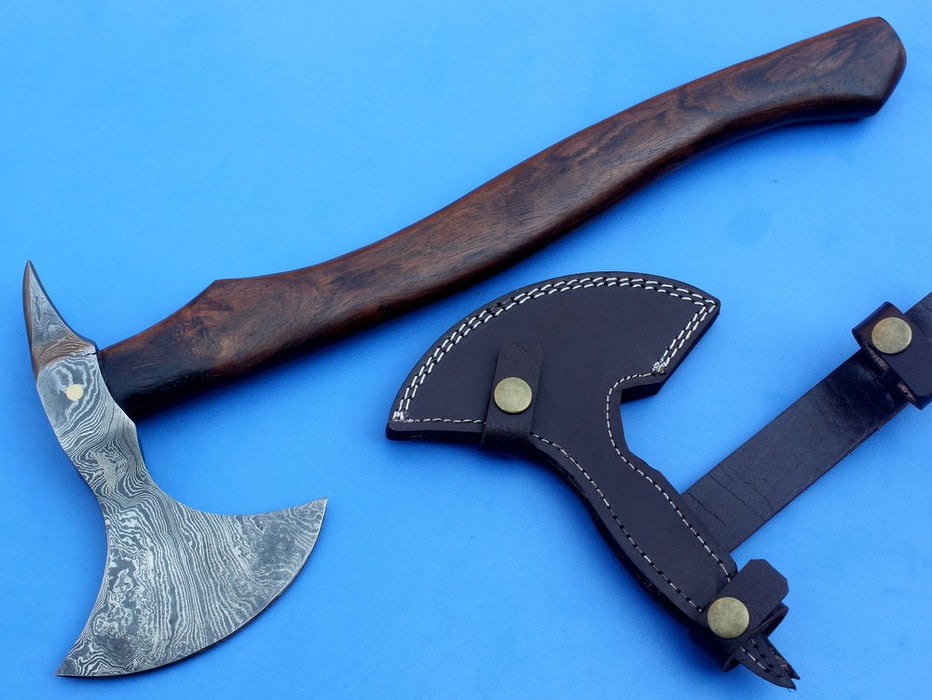This is a detailed image featuring a small, new axe with a medium-sized, dark wooden handle that extends from the top-right corner to the bottom-left corner of the frame. The handle has black accenting, and the sharp-edged metal blade rests at the lower-left portion of the image. The background is a bright periwinkle blue, providing a vibrant contrast to the axe. Positioned close to the axe, in the bottom-right corner, is a black holster, designed to fit the axe's shape perfectly. The holster is equipped with three circular snaps or buttons—one at the end of the blade, one at the front, and one near the middle where it would secure the handle. The holster's design is adorned with little buckles, possibly gold, emphasizing a custom fit for the irregularly shaped blade. The composition of the photograph is clear and simple, with no text or people present, focusing solely on the axe and its accompanying holster.